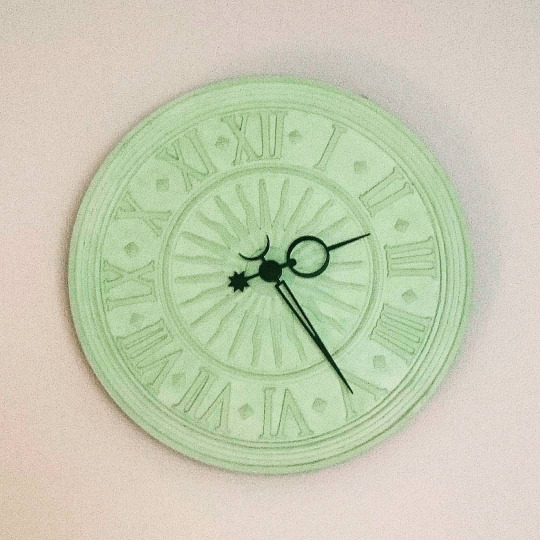This wall clock is a serene pale seafoam green, reminiscent of a gentle ocean breeze. Expertly crafted, possibly from resin or ceramic, it features a smooth matte finish that exudes a subtle elegance. Intricately designed Roman numerals mark each hour, seamlessly integrated into the casting. Central to the clock's face is a radiant sun motif, with rays extending outward in a captivating pattern. The clock's hands, starkly black against the green backdrop, are uniquely shaped as celestial symbols—a star, a crescent moon, and a circle representing the sun—adding an artistic and whimsical touch to this timeless piece.